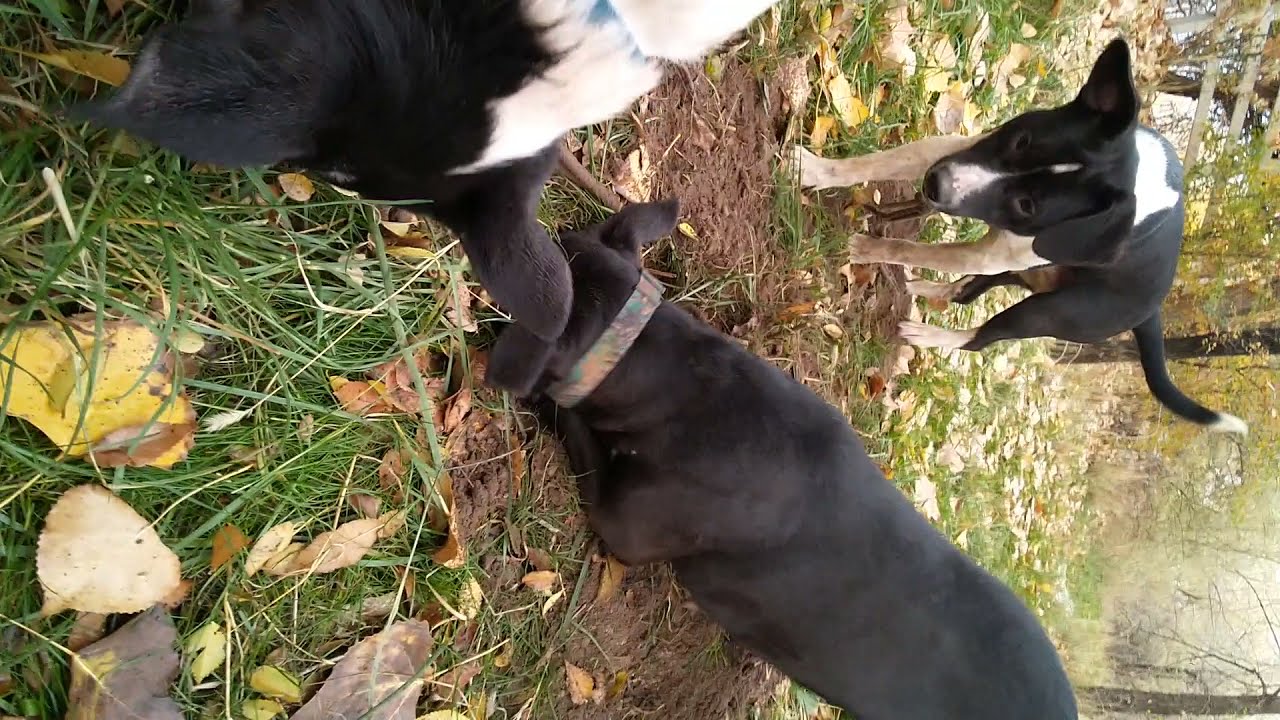This captivating, slightly tilted portrait photograph depicts three playful young dogs deeply engaged in an outdoor adventure in a forest setting, suggesting a crisp autumn day with fallen yellow and brown leaves scattered across the grass-covered ground. The central focus is a black dog energetically digging into a dirt hole, possibly hunting for a rabbit, with its head fully immersed in its pursuit. Positioned closely behind, a second black-and-white dog, characterized by its white legs and lifted tail, seems eager to join the excavation. Meanwhile, in the foreground, the slightly blurry head and neck of a third dog, also black-and-white, peek into the frame, curious and eager to be part of the action. The scene radiates a sense of wild, doggy fun and exploration, unaccompanied by any humans, highlighting the dogs' natural instincts and camaraderie.